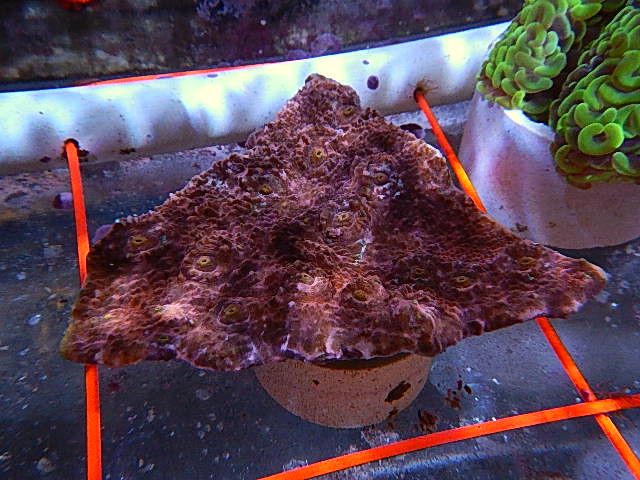The image shows a peculiar triangular-shaped brown fungus or aquatic plant with a rough and bumpy surface, marked by small yellow circles and white patches. It appears to be growing from a tan or light-colored pot resembling concrete, resting on a gray concrete floor. Surrounding the plant is a neon orange piping or wire barrier that emerges from two holes in a white curb-like structure, forming a protective enclosure around the specimen. To the right, another green aquatic plant with C-shaped or U-shaped leaves sits in a concrete planter. Both plants seem to be part of an experimental setup, possibly in a lab or specialty store dedicated to unusual plants. The scene is scattered with some dirt and debris, suggesting an environment focused on scientific research or conservation efforts.